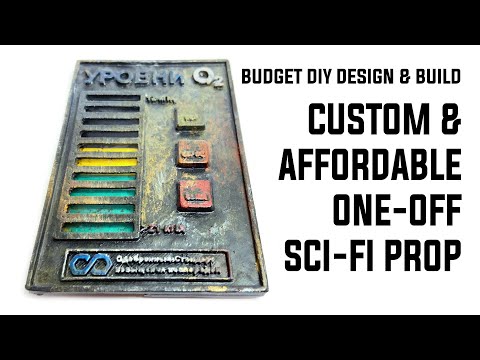The image appears to be a screenshot from a video, characterized by black bars at the top and bottom, and a central white background. On the left side, there's a metal sci-fi prop, possibly used in movies or plays. This prop features Cyrillic text and the letters "Q2" or "O2" at the top right, suggesting a sci-fi theme, perhaps related to oxygen. The prop is detailed with rectangular slats, five of which are gray, followed by two yellow slats and four green slats. Additionally, there are small, dusty-looking buttons or raised squares and an infinity symbol with more unreadable text at the bottom. On the right side of the image, bold capitalized text reads "Budget DIY Design and Build," followed by "Custom and Affordable One-Off Sci-Fi Prop" in larger text. The prop overall has a meticulously detailed, handmade appearance emphasizing its custom and budget-friendly nature.